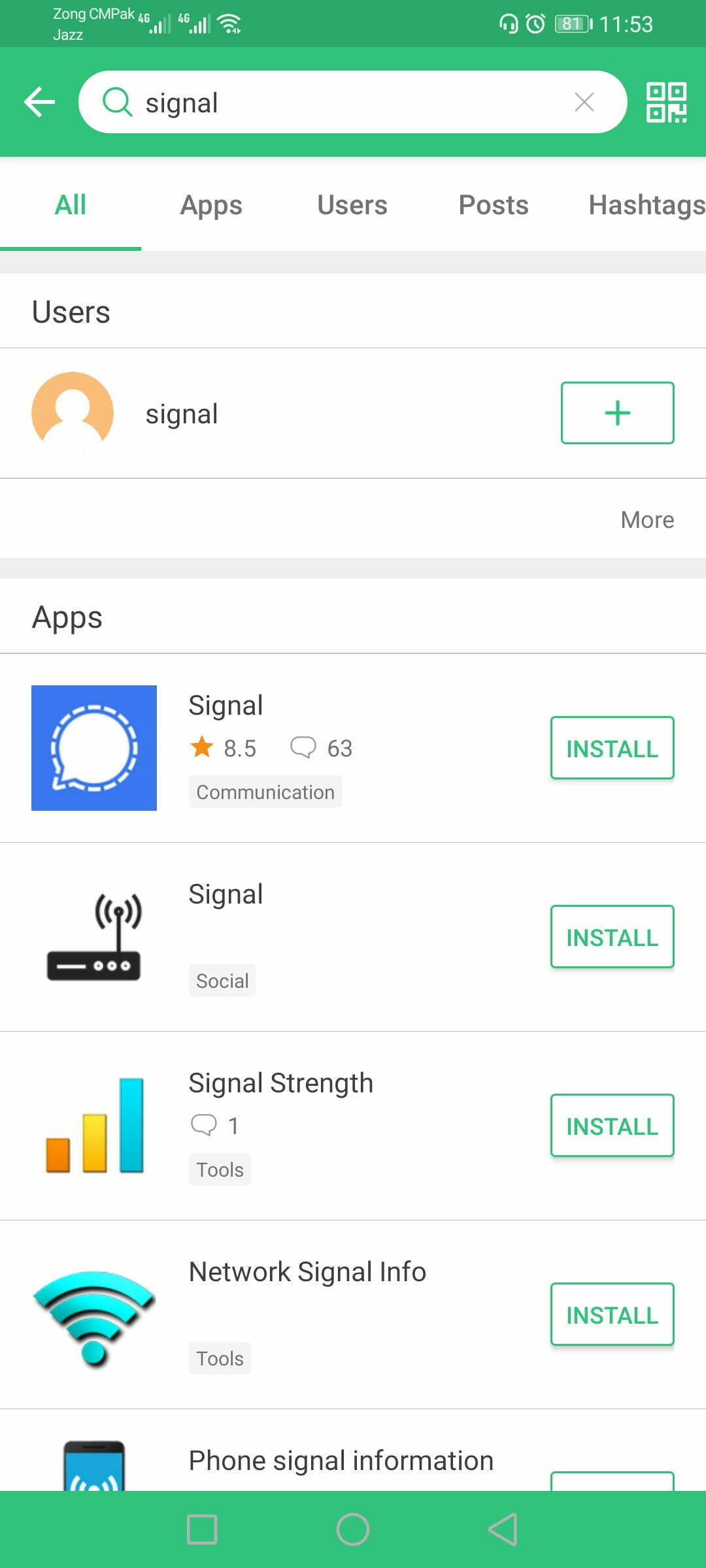The image showcases a mobile app store search interface, featuring a predominantly green theme. At the top, there are two banners in varying shades of green, with the uppermost banner in a darker hue. The upper banner displays the text "ZONG SMPAK" followed by "Jazz" beneath it. On this banner, there are three different signal strength icons and various cell phone indicators on the right, including the time (11:53) and battery life (81%).

Below these banners is a green box containing a white search field where "signal" has been typed in. Tabs labeled "All," "Users," and "Signal" allow for search categorization, with "All" currently selected. A list of apps relevant to the keyword "signal" is shown underneath. Each app entry includes its name, rating out of 8.5 stars, and number of comments. Examples of the listed apps are "Signal," "Signal Strength," "Network Signal," "Signal Info," and "Phone Signal Information." To the right of each app's name is a green-bordered rectangle with the word "Install," indicating the option to download the app. The context suggests the user is searching for an app to gauge their phone's signal strength.